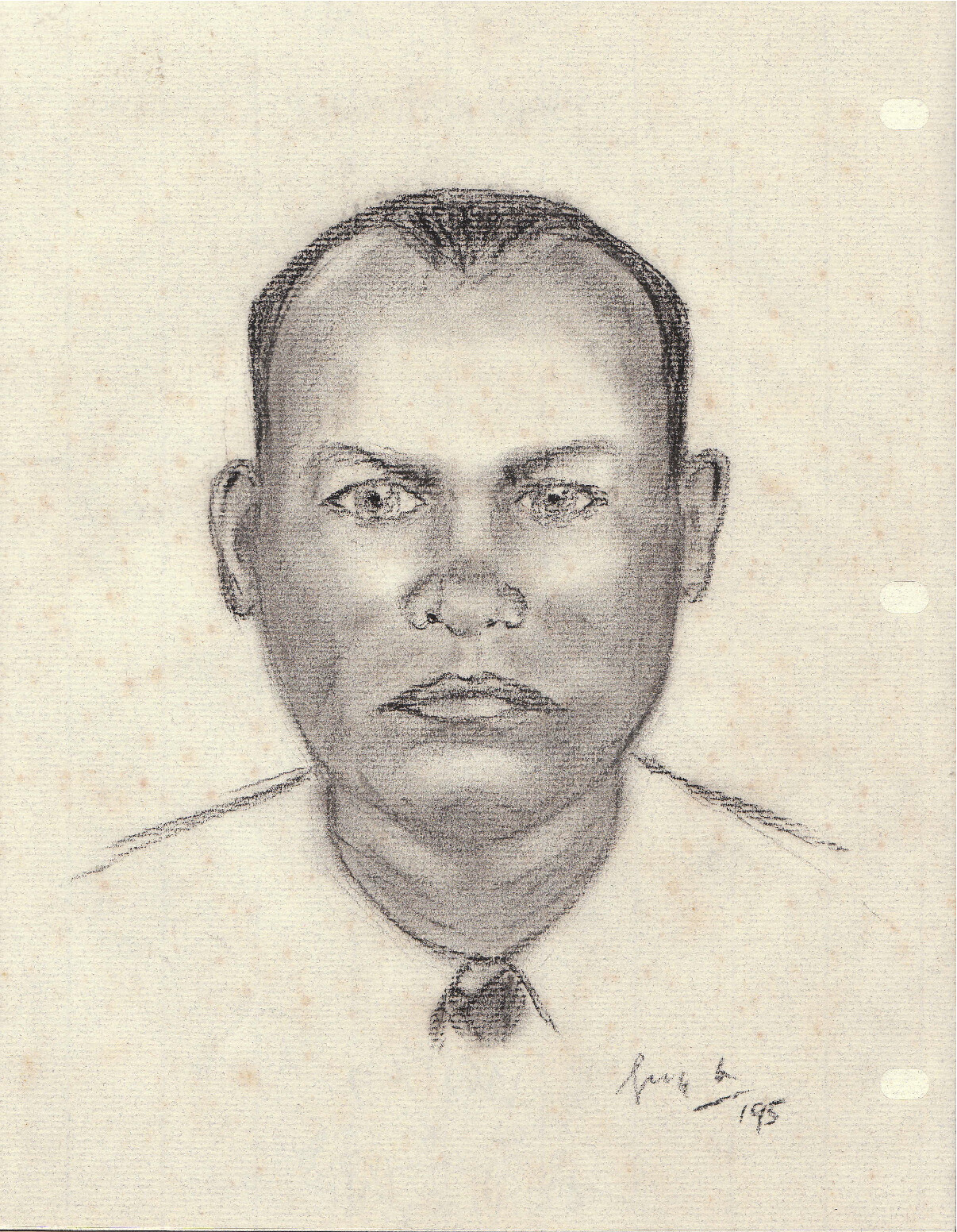This detailed sketch depicts the head and upper neckline of a man, extending down to the beginning of a tie. The man's face is shaded to suggest a dark skin tone, and he has short, dark hair that is depicted with even heavier shading than the face. The hairline is noticeably receding at the top. Around the eyes, the artist employed a much lighter tone, with minimal shading, to accentuate the dark eyebrows and light-colored eyes. Only the upper parts of the shoulders are sketched, alongside a clearly defined neckline and what seems to be a white and black tie, although the precise colors are indeterminable due to the black and white nature of the sketch. 

A partially legible signature appears at the bottom of the image, along with a potential initial that looks like 'G'. The first letter of the name appears to be 'R' or 'L', but it is indistinct. Beneath this, there is a dashed line followed by the number "195." The sketch is drawn on yellowed paper, indicating its age.